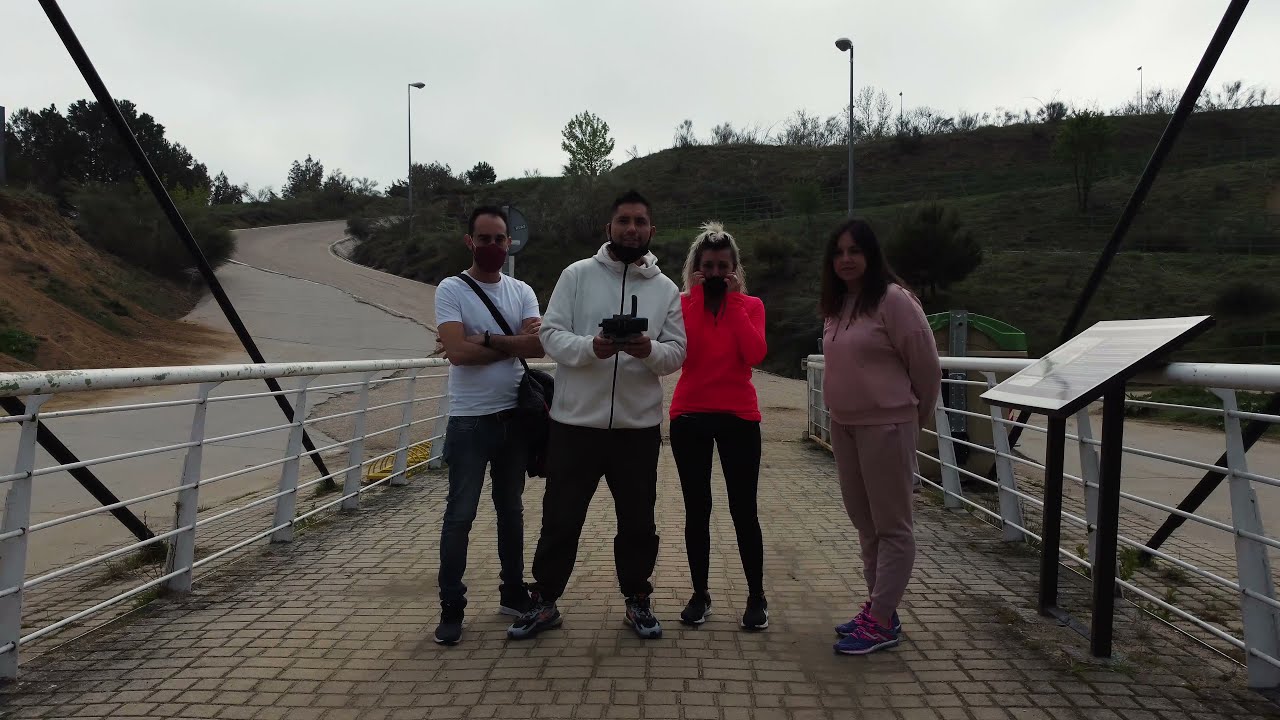This image captures a group of four people standing on a concrete or brick walkway, likely a bridge, with white steel railings on both sides. The railings consist of a white steel pole at the top with several smaller lines underneath. The bridge is supported by white pillars. In the background, a winding road curves around rocky, grassy hills. The overcast sky adds a grayish-blue hue to the scene. The bridge also features black wires and light posts.

From left to right, the people are dressed as follows: The first man, with short dark hair and wearing glasses and a maroon face mask, sports a white t-shirt, blue jeans, and tennis shoes. The second man, with a dark beard, wears a white hoodie, dark pants, and tennis shoes. The third individual is a woman with blonde hair, wearing dark pants and tennis shoes, and appears to be holding something near her face. Finally, the fourth person is a woman dressed in a cream-colored shirt and pants with tennis shoes and has long dark hair. Adjacent to them, there's an unreadable sign held up by black posts.

The setting and attire of the individuals suggest that it might be fall. The overall mood is calm and somewhat muted due to the cloud-covered sky.